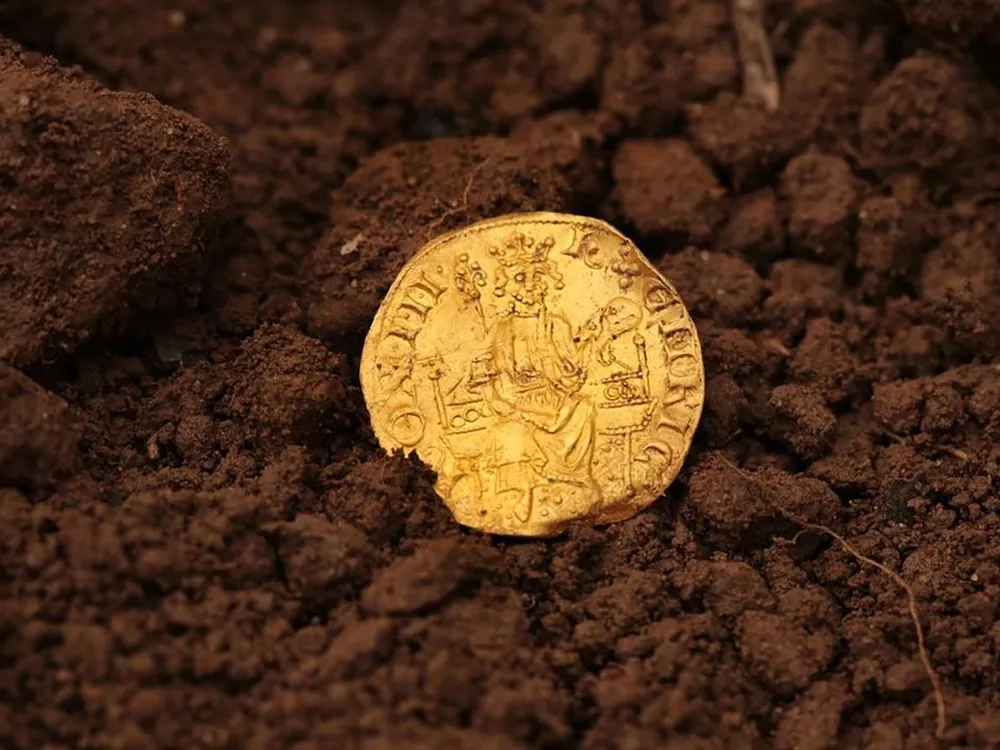A close-up image showcases an ancient, golden coin partially embedded in coarse, earthy soil. The background and foreground are dominated by rich, textured dirt, revealing clumps, tiny specks, and even a small root fiber. The central focus is the coin, a roughly circular artifact that clearly dates back to pre-industrial times, as evidenced by its irregular, wobbly edges. The coin features an intricately detailed image of a robed king, complete with a crown and scepter, seated on a throne-like bench. Encircling the figure are inscriptions in an unknown language, possibly Latin, with a discernible Roman numeral "III." The coin's weathered appearance underscores its historical significance, making it a fascinating find amid the mundane soil.